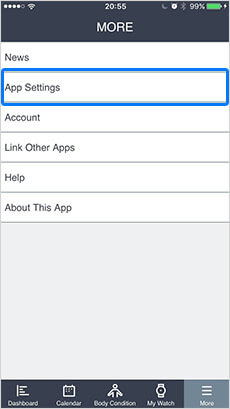A screenshot of an application's interface, specifically from the "More" section, with the word "MORE" displayed prominently in all caps at the top in black. Below this heading are several selectable options: "News," "App Settings," "Account," "Link Other Apps," "Help," and "About This App." The "App Settings" option is currently highlighted with a blue outline around the entire box, indicating it is selected. At the bottom of the screen, a navigation bar includes icons labeled "Dashboard," "Calendar," "Body," "Coronation," "My Watch," and "More." The "More" icon at the bottom right is shaded in gray, signifying the user is currently in this section.